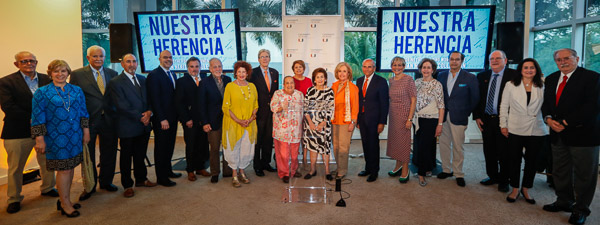This photograph, taken indoors, showcases a diverse group of approximately 20 people composed of both men and women. The men, predominantly in their mid-50s and older, are all dressed in dark suits and ties, exuding a formal and distinguished appearance. The women, on the other hand, are elegantly attired in a mix of colorful dresses, skirts, and a few in pant suits. Everyone is smiling at the camera, giving the scene a warm and welcoming feel.

The group is positioned on brown-colored flooring, lined up neatly from left to right. At the front of this lineup is a clear acrylic pedestal, suggesting that this might be a formal event where someone will likely make a speech. The background features two TV screens that display "Nuestra Herencia" in blue writing. Flanking these screens are some speakers, likely for audio support.

Adding to the ambiance of the setting are large glass windows behind the group, offering a view of what seems to be a tropical locale with visible palm trees and possibly some water. This detail enhances the impression that this event is taking place in a scenic and sunny environment.